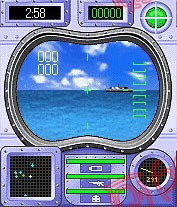The image is a detailed artistic graphic, likely a screen capture from a video game, depicting a complex control panel with a central viewport. The background of the interface is purple, with darker shades at the bottom and lighter at the top. In the middle of the view, through what appears to be a binocular or submarine-like window, the horizon of an ocean is visible, featuring a large ship with white structures sailing sideways from left to right. The sea is a blend of blue with a hint of green, while the sky above is a clear blue adorned with white clouds.

Surrounding the central viewport are various digital readouts and dials. At the bottom left corner, there is a radar-like display with blue and white dots. Symbols representing a battery, a gun, and a building are visible in green. Additionally, there are numerical readings: the number 258 appears in white at the top, while 000 and a green circle with a white cross are situated nearby. The overall interface is adorned with green markers and rectangular information boxes, which likely indicate levels, distances, and other game-related metrics. The entire setup vividly mimics the immersive experience of navigating a high-tech virtual environment.